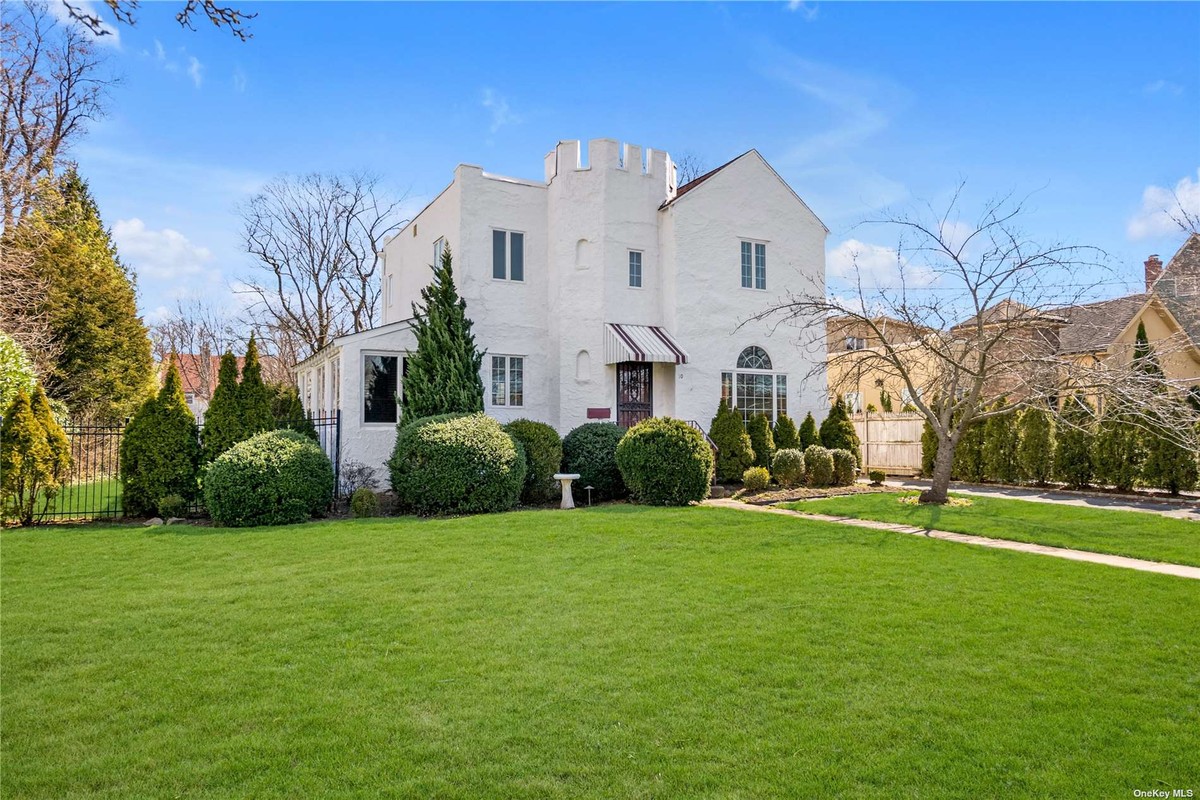This photograph depicts a well-maintained two-story house with a uniquely designed center structure resembling a castle tower. The exterior features a stone-white siding, and the central part rises prominently, adorned with decorative elements reminiscent of a chessboard pattern. The roof includes normal peaks on either side of this castle-like structure.

The home's front entrance is characterized by a large iron gate screen and an awning overhead, providing both aesthetic appeal and practical shelter. Below the awning, a decorative door invites entry, flanked by a total of three windows on the second story, emphasizing symmetry and elegance.

The meticulously manicured lawn in the foreground showcases the care given to the landscape, featuring neatly trimmed shrubbery and round bushes, as well as a small fountain. A walkway extends from the front door through this vibrant green grass to the edge of the frame. The scene suggests a fall setting, with trees in the background displaying yellowing leaves or standing bare, adding a touch of seasonal charm.

In this bright, daytime photograph, the sky is a beautiful light blue with scattered white clouds, contributing to the serene and picturesque setting of this distinguished home.